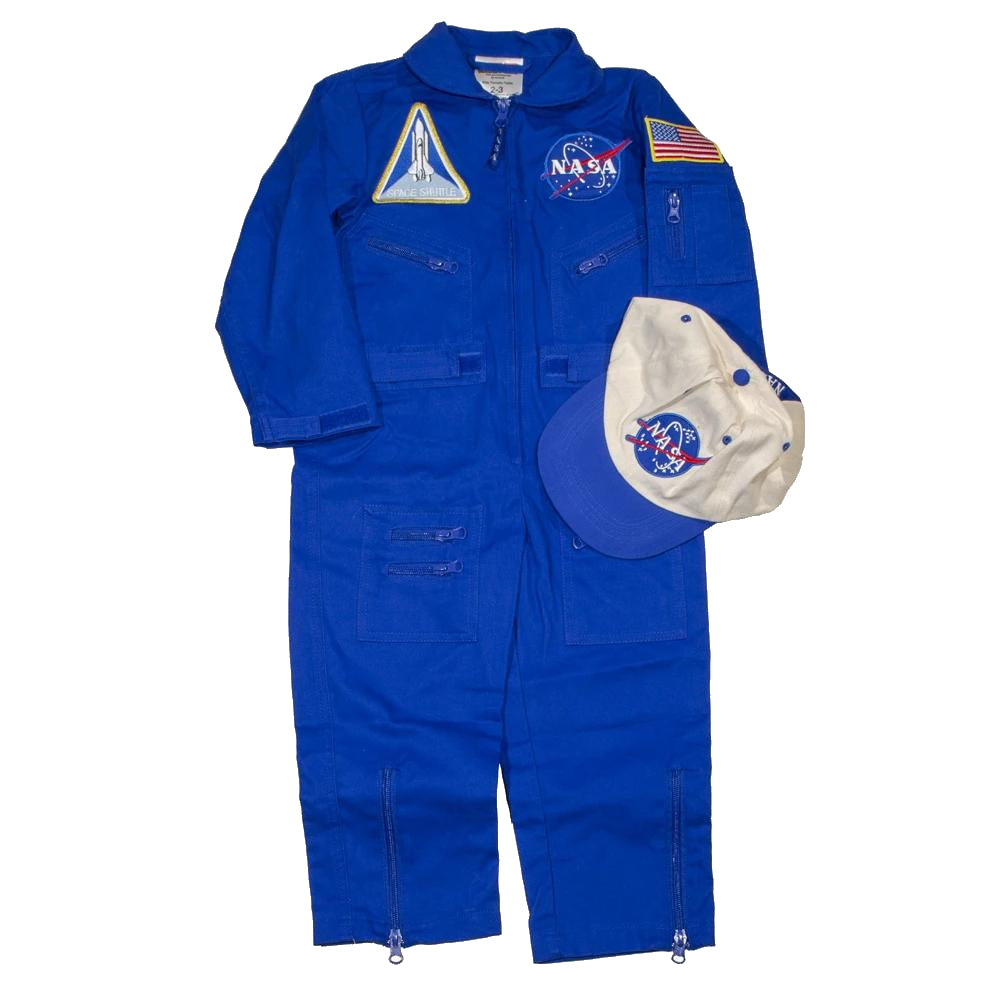The image showcases a vibrant blue children's astronaut costume set against a clear white background, giving it a stock photo appearance. The costume is a detailed one-piece jumpsuit complete with long sleeves and legs, featuring two front diagonal zippers on the chest and additional zippers on each leg extending from the cuff to the knee area. The design is adorned with three distinct patches: a triangular patch depicting a space shuttle on the left breast, a circular patch with the NASA logo on the right breast, and an American flag patch on the left sleeve. To complete the ensemble, a white baseball cap with a blue brim and the classic NASA logo is included. The costume has practical elements such as buckles, snaps, and pockets on each leg, and it is characterized by a prominent collar, making it a detailed representation suitable for a Halloween costume or imaginative play.